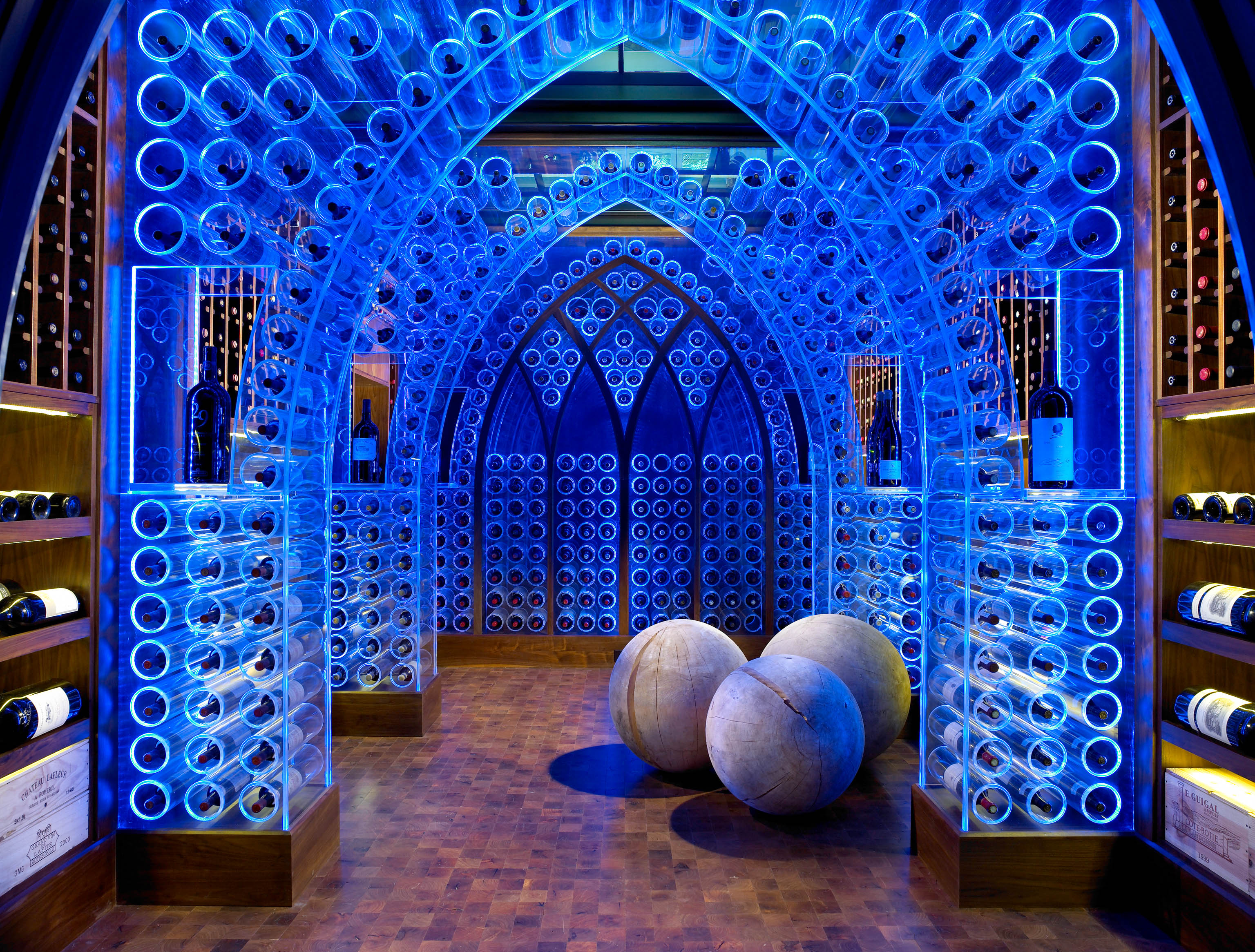This photograph captures a striking and unique wine cellar with a distinctly modern and futuristic aesthetic. The scene is set in a hallway framed by traditional wine storage areas along the left and right walls, featuring typical brown wooden shelves lined with wine bottles. Dominating the center of the hall are several arch structures constructed from blue-tinted glass or acrylic, emitting a cool, illuminated glow. These arches have a Gothic shape with pointed tips and contain compartments and rectangular openings for storing wine bottles, which lie both horizontally within circular slots and vertically in the cutouts. The floor of the cellar appears to be made of brown wooden tiles, adding a warm, classical touch. Additionally, the room features three large wooden spheres on the ground, lending an intriguing element to the overall decor. The combination of conventional wooden cabinets and innovative glass arches, with bottles elegantly displayed within, makes this wine cellar both avant-garde and visually captivating.